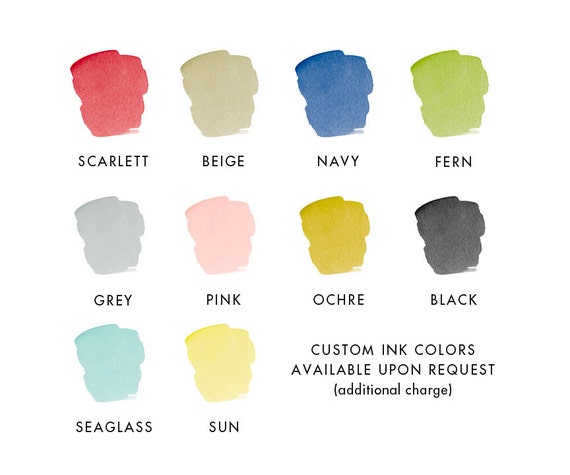The advertisement showcases an array of custom ink colors neatly arranged on a pristine white background. The colors are displayed in three rows, with four splotches each in the top two rows and two in the bottom row. Starting from the top left, the first row features a vibrant scarlet accompanied by its label in black text, followed by a beige splotch labeled "beige," then a deep navy labeled "navy," and finally, on the top right, a light green labeled "fern." The second row from left to right begins with a subtle gray labeled "gray," a lively pink labeled "pink," a rich ochre labeled "ochre," and a bold black labeled "black.” The bottom row includes a refreshing light blue labeled "sea glass" on the left and a sunny yellow labeled "sun" to the right. In the bottom right-hand corner, the text "Custom Ink Colors" is prominently written, with a note underneath stating "Available Upon Request" and an additional mention that there is an "additional charge" for these custom colors. This detail-oriented presentation emphasizes the variety and availability of unique ink colors for customization.